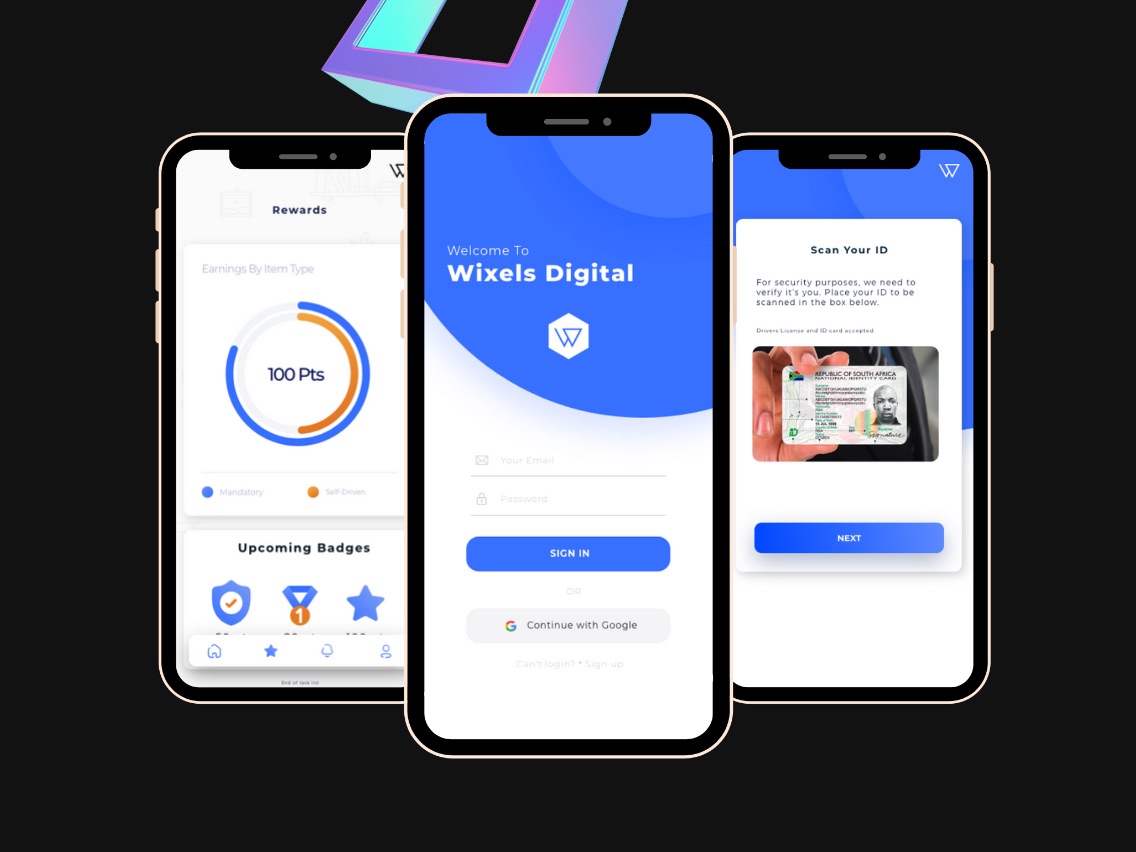This digital photograph features a stark, black background that artfully contrasts with the vibrant elements at the center. Dominating the composition is a thick, 3D-ish square placed in the upper center, radiating gradients of light green, purple, and pink. Below this vivid frame are three smartphones arranged in a linear formation, each displaying distinct screens within three columns.

In the leftmost column, the smartphone screen displays a rewards interface. The interface includes an outlined phone frame with three buttons on the left. The screen prominently features the text "Rewards" followed by a spacious white content area titled "Earnings by Item Type." Within this area, a bold "100 points" is encircled by dual rings—one blue, labeled "mandatory,” and one orange, labeled "self-driven." Beneath this segment are the upcoming badges: the first badge resembles a shield with an orange check mark, the second appears as a ribbon with a "1" inscribed within a circle, and the third badge resembles a blue star. Below the badges is a row of familiar icons: a home icon, a blue star, a notifications bell, and a person icon.

The central column focuses on a welcoming screen for "Wixels Digital," with the name "Wixels" spelt out in bold letters. The background transitions smoothly from a solid blue to a lighter blue towards the upper right corner. The brand’s logo, featuring a line curving downward and upward adjacent to a triangle, is prominently placed below the welcoming message. The screen prompts users to enter their email and password, offering a primary blue "Sign In" button with an alternative option to continue with Google.

The rightmost column highlights a straightforward instruction: "Scan your ID," followed by a "Next" button. This prompt signals the next step in the process, indicating a streamlined and user-friendly interaction.

Together, these elements create a dynamic and visually engaging narrative, showcasing a blend of functional design and vibrant aesthetics.